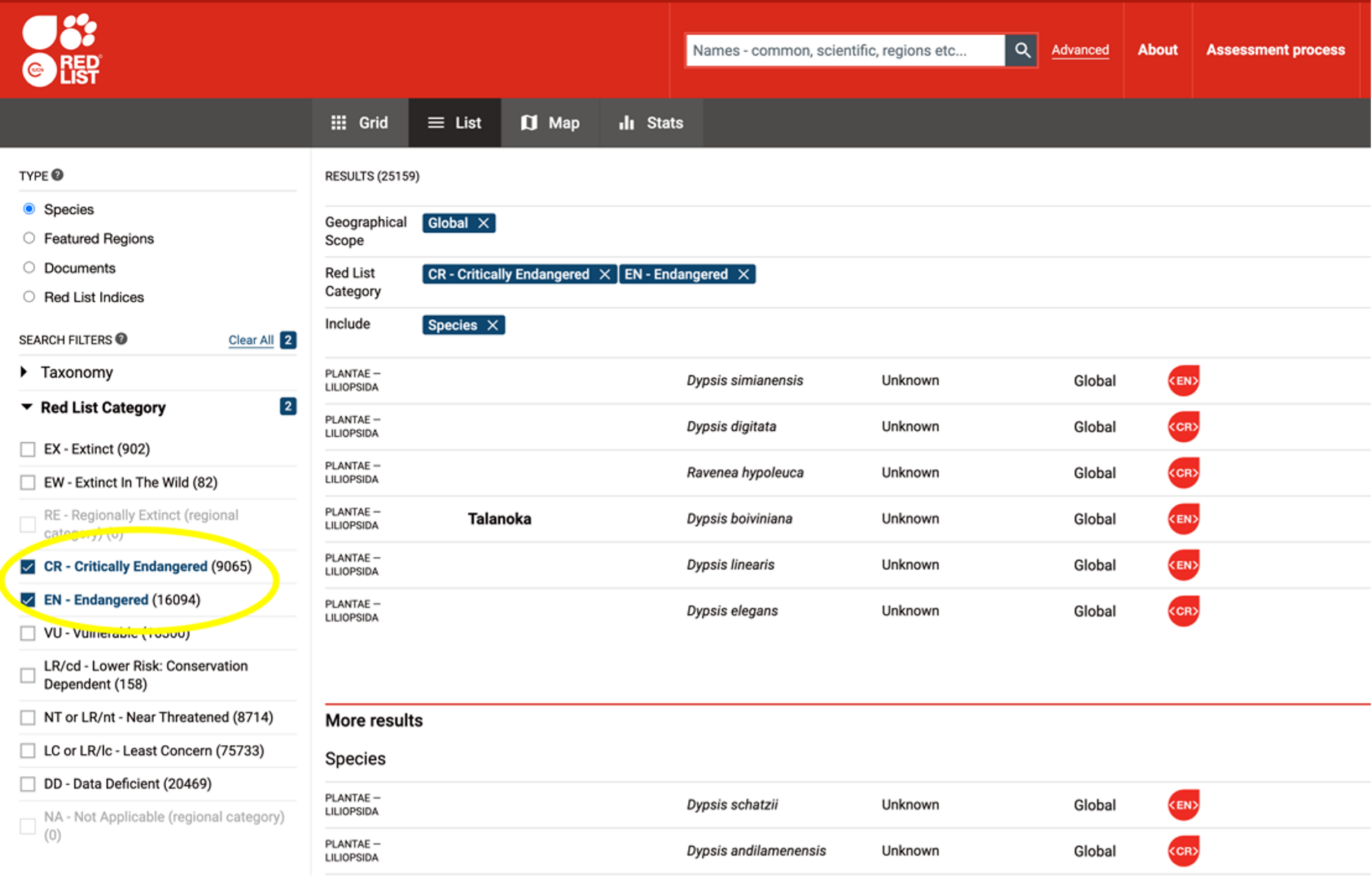The webpage showcases a detailed and informative interface dedicated to the Red List. In the upper left-hand corner, there is a distinct logo labeled "Red List," featuring various elements, including a foot, a paw print, a water drop, and other symbols on a red background. 

A search bar prominently sits next to the logo, equipped with placeholder text such as "Names, Comments, Scientific, Regions, etc." To its right are several navigational links in white text, including "Advanced," "About," and "Assessment Process."

Below this primary header is a secondary navigation bar with options labeled "Grid," "List," "Map," and "Stats," each accompanied by relevant icons—a grid icon, a hamburger menu icon, a map icon, and a graph icon, respectively. This secondary bar is characterized by its gray background and white text and icons.

The main section of the page displays a comprehensive list of items organized into multiple columns, detailing various types of information. On the left side of the page, occupying approximately 20% of the space, is a sidebar with a range of selectable options, including "Type," "Species," "Featured Regions," and "Documents," along with radio buttons for selection.

Further down the page, there's an extensive array of search filters, covering categories like "Taxonomy," "Red List Category," and specific statuses such as "Critically Endangered." The primary portion of the page displays the search results, indicating filtered criteria such as geographical scope and species categories. The results feature both common and Latin names, highlighting various species and plants.